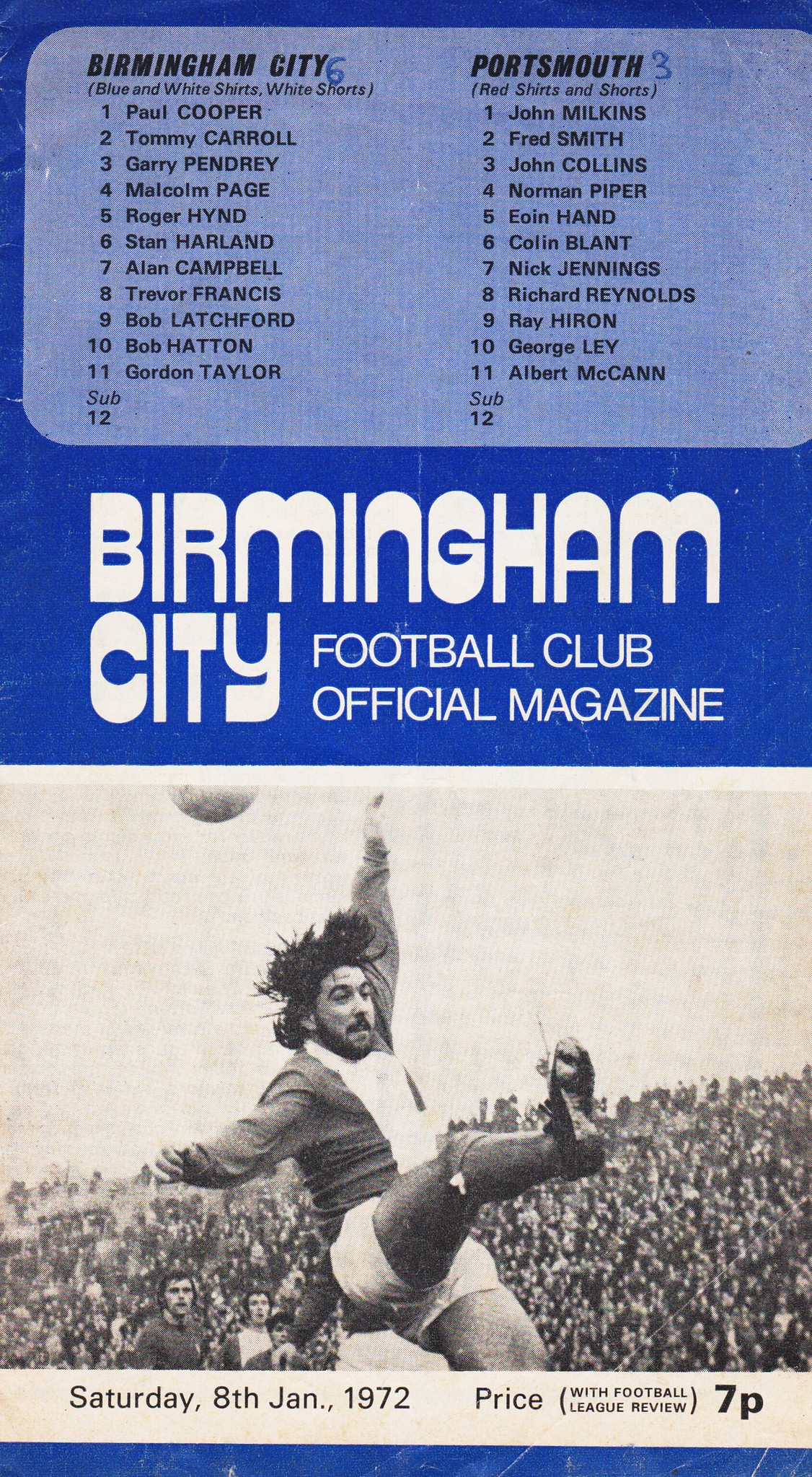The cover of the Birmingham City Football Club official magazine is divided into two distinct sections. The upper half features a dark blue background with a light blue inset at the top, which is a horizontal rectangle with rounded corners. This inset contains two columns of text listing the team players for Birmingham City and Portsmouth. The left column is headed "Birmingham City" and lists players with described uniforms of blue and white shirts with white shorts, including names such as Paul Cooper and Trevor Francis. The right column, headed "Portsmouth," lists players with red shirts and red shorts, including names like John Milkens and Fred Smith.

Just below this inset, on the dark blue background, "Birmingham City" is prominently displayed in bold white lettering, followed by "Football Club Official Magazine" in smaller white text. 

The lower half of the magazine cover is dominated by a striking black-and-white photograph. The image captures a dynamic moment of a soccer player in mid-air, his right leg extended forward as if he has just kicked a ball, which is visible above his head. The player's left arm is raised upward for balance while his right arm extends outward. He has dark hair, a full mustache, and beard, and wears a jersey with a distinguishable white stripe down the center, along with white shorts. 

In the background, a stadium full of spectators watches intently, adding a lively ambiance to the scene. 

At the bottom of the cover, a white bar with black text reads "Saturday, 8th January, 1972" with the word "Price" followed by the phrase "(With Football League Review)" and "7p" printed in bold. Just below this, a horizontal bar of dark blue, matching the upper part of the cover, completes the design.